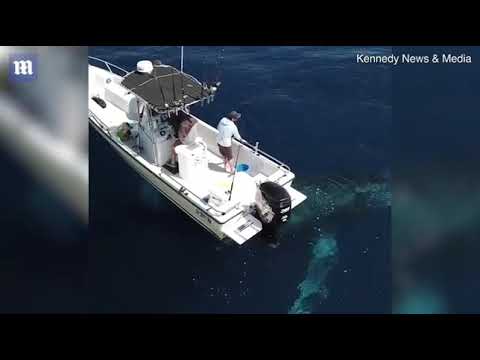The image captures a small white fishing boat with a gray canopy situated in a dark blue ocean, brightly lit by the sun. The boat is at the center and slightly right of the frame, with its bow pointing toward the upper left corner. A man, wearing a white t-shirt, grayish hat, and off-red shorts, stands on the boat, looking over its starboard side. The stern features a prominent black outboard motor, and near it, in the water, there's a faint silhouette of a large fish or possibly a shark. The photograph has a blurred background on both sides and is bordered by thin gray vertical rectangles. Across the top right corner, there’s a watermark reading "Kennedy News and Media" in white lettering, along with an "M" logo inside a dark blue box on the top left. The image is enclosed within black borders at the top and bottom.